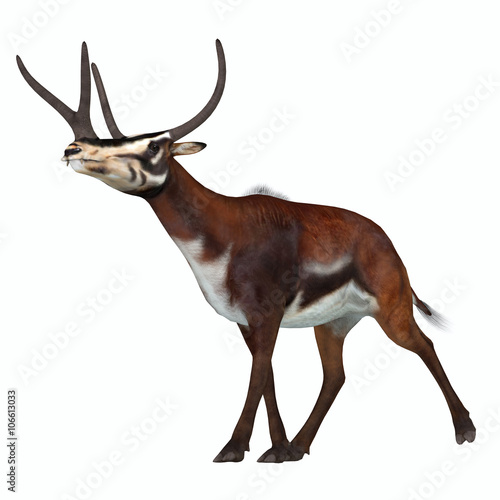The image depicts a detailed sketch of a large mammalian herbivore known as Kyptoceras. This prehistoric animal, an antelope-like mammal from North America during the Miocene and Pliocene periods, is positioned against a white background, giving a clear view of its features. The creature possesses a body resembling that of a large caribou or elk, yet with distinctive characteristics. Its head is a mix between a cow and a horse, featuring large, two-pronged horns forming a shape reminiscent of the letter Y. The animal is primarily brown, with an off-white face, chest, and underbelly. The face includes brown markings around the eyes and some striped patterns beneath them. It is depicted in a walking stance, with its head held high and one front leg stepping forward while the back leg is trailing behind. The Kyptoceras has black hooves, a short brown tail with a white tip, and a mane-like patch of hair at the shoulders. Overall, the sketch captures the unique and somewhat ominous appearance of this ancient mammal.